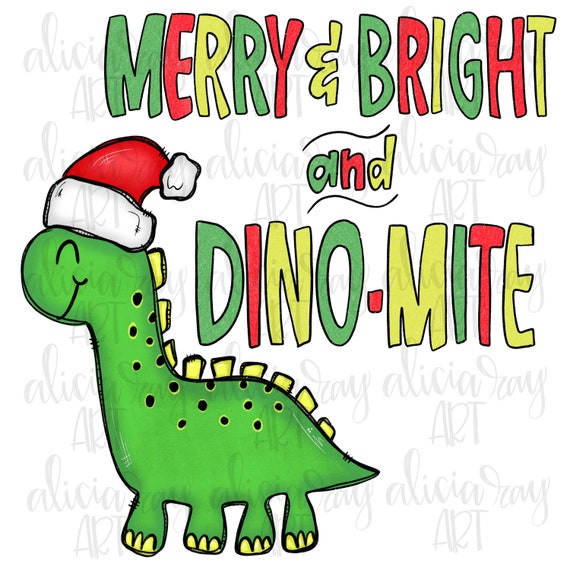This image is a hand-drawn illustration, reminiscent of a children's comic book cover or a Christmas card. Dominating the top section, whimsical text reads “Merry and Bright, Dino-Mite” in alternating colors of green, red, and yellow, adding a festive, playful touch. Positioned in the lower-left corner is a cartoonish, long-necked dinosaur with a green body dotted with black spots and adorned with yellow spines along its back. The dinosaur is festively dressed in a Santa hat, characterized by a red cap, a white brim, and a fluffy white pom-pom at its tip. The entire scene is set against a plain white background, marred slightly by an unclear repeating watermark.